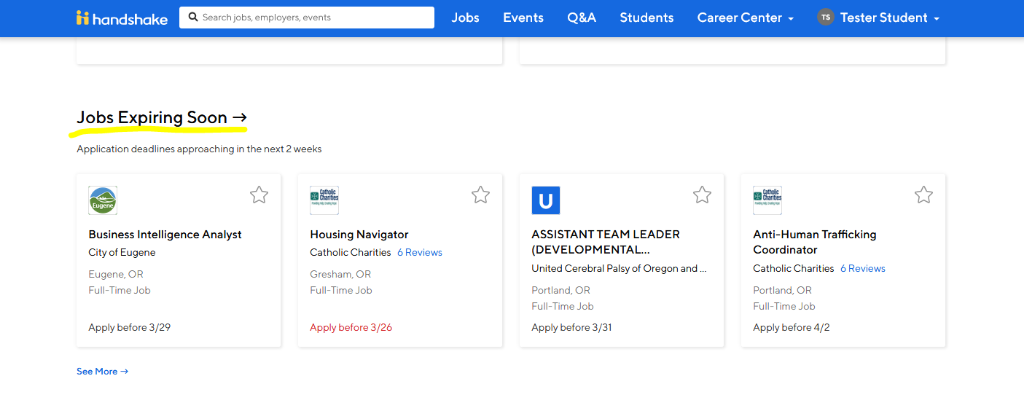The image shows a webpage on the platform Handshake, featuring a well-structured user interface designed to assist users in navigating job-related resources. At the top left corner, a search bar is prominently placed, allowing users to search for jobs, employers, and events. The top navigation area, set against a blue background, includes tabs for Jobs, Events, Q&A, Students, Career Center, and a section presumably still under development labeled Test Your Student.

On the main page, a highlighted section titled "Jobs Expiring Soon" draws attention. This section, marked by an added underline in highlighter, emphasizes the urgency of upcoming application deadlines within the next two weeks. Underneath this heading, several job listings are provided, including roles such as Business Intelligence Analyst in Eugene, Oregon; Housing Navigator in Gresham, Oregon; Assistant Team Leader in Portland, Oregon; and Anti-Human Trafficking Coordinator, also in Portland.

Each listing notes the respective expiry date of the job application period. One particular listing has its deadline highlighted in red text, urging applications before March 26th, indicating an immediate deadline. The latest deadline mentioned is for a job expiring on April 2nd.